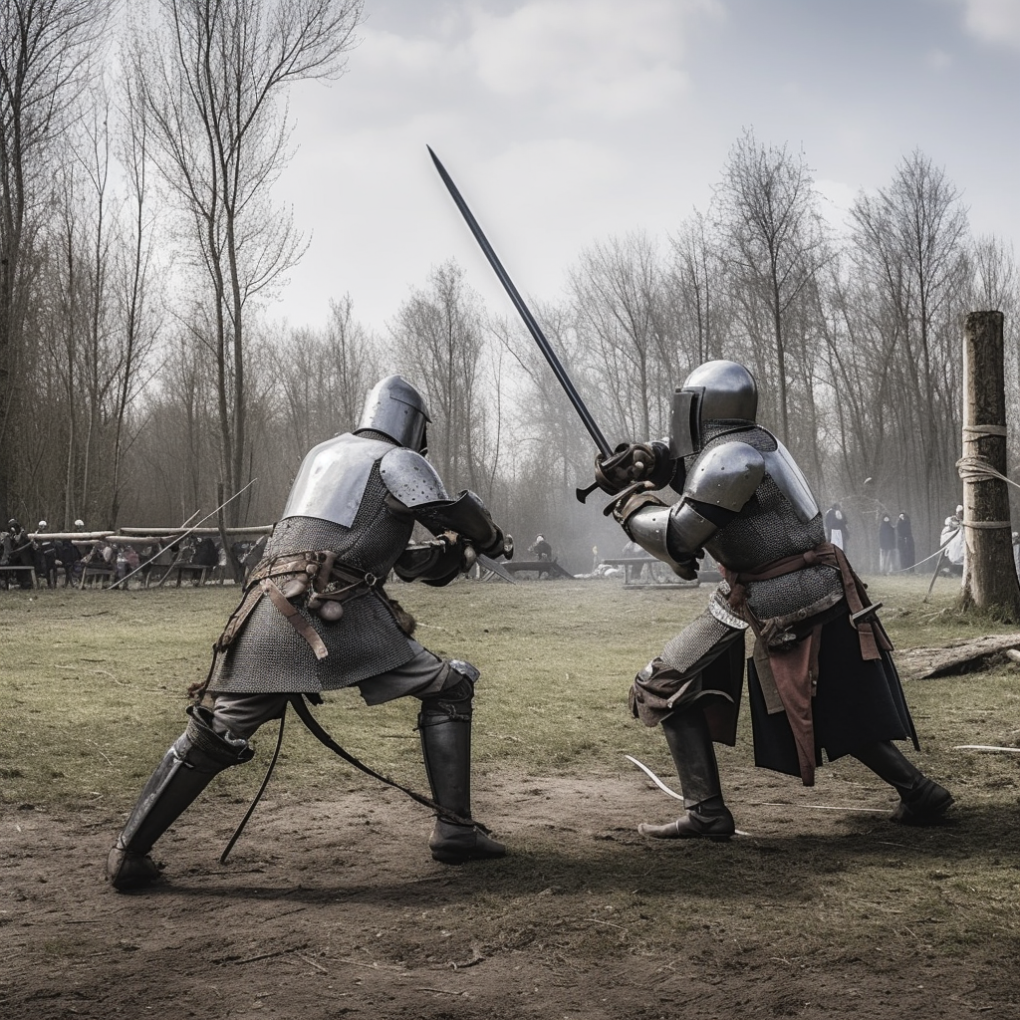The photograph depicts a dramatic scene of two medieval knights engaged in battle, set against an outdoor backdrop. Both knights are fully clad in intricate armor, which includes steel helmets, shoulder plates, and chain mail covering most of their bodies. The knight on the center-right is captured mid-swing with a long, vertical steel sword held with both hands, poised to strike. His armor includes a mix of steel plates on the upper body and chain mail below, complemented by brown and black cloth accents, including a brown leather belt and knee-high black boots. On the center-left, the opposing knight mirrors this attire, with similar steel and chain mail armor, but with his sword partially obscured as it is outstretched to the side.

In the background, one can discern the chaos of a larger battlefield, where half a dozen blurred figures are seen fighting. Dominating the scene are tall, leafless trees with numerous thin branches, which extend up into a sky washed in blue with patches of white clouds and some mist. A notable feature is a 10-foot-high tree stump to the right, adorned with ropes, suggesting a rugged and untamed setting.

The ground beneath the combatants is a mix of dark brown dirt and patches of short, light green grass, hinting at a late autumn atmosphere. Additional details include brown leather pouches attached to the knights' belts, presumably for carrying essentials, and more soldiers and equipment scattered deeper in the scene, faintly visible through the haze. The overall visual composition suggests a scene that might be enhanced with CGI or AI for a rich, cinematic effect.